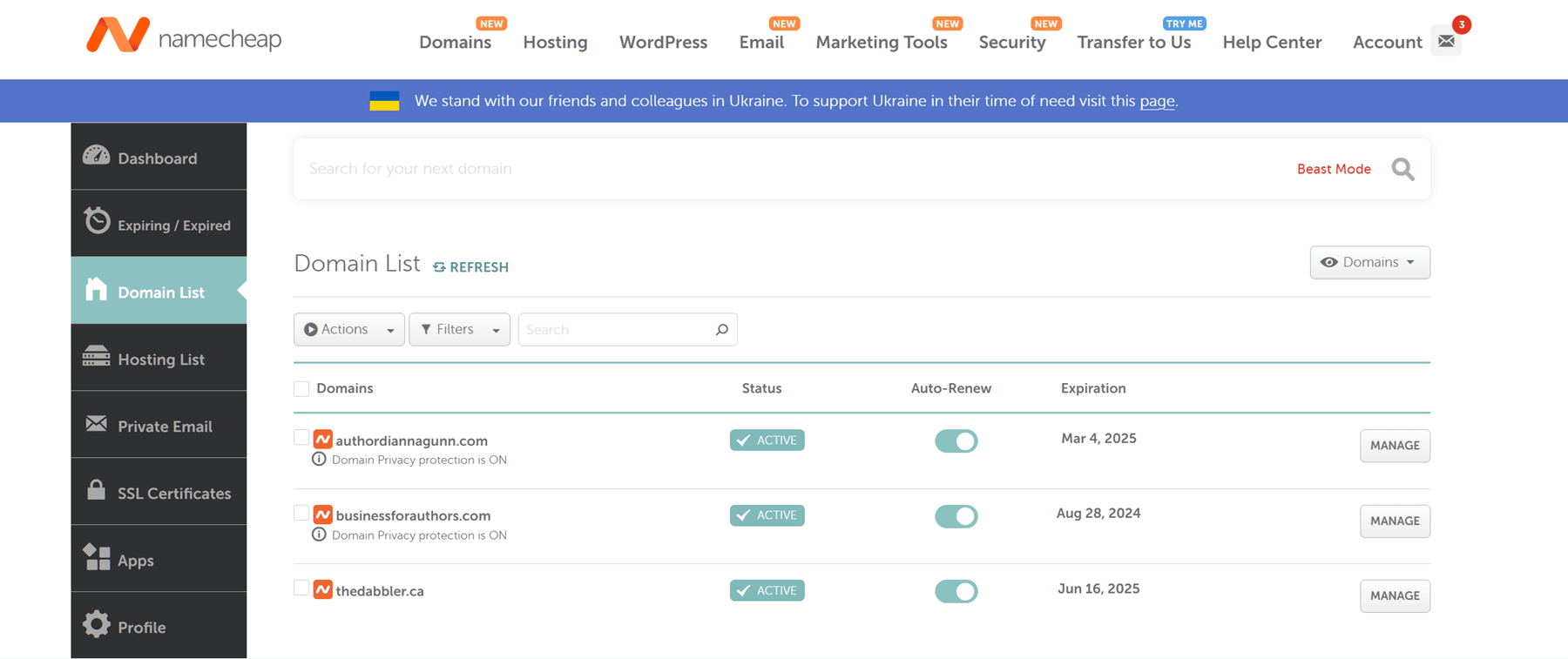### Detailed Caption for the Namecheap Website Image

The image is a screenshot of the Namecheap website's interface. In the top left corner, there is a stylized "N" logo featuring shades of orange; the tip is dark orange, the middle is a lighter orange, and the bottom returns to a darker orange. To the right of the logo, the word "namecheap" is written in a very light black, lowercase font without any spaces.

Moving towards the right, a main menu appears with several options:
1. **Domains** - Marked with an oval, orange "New" icon in white text at the top right.
2. **Hosting**
3. **WordPress**
4. **Email** - Also marked with the "New" icon.
5. **Marketing Tools** - This option has the "New" icon as well.
6. **Security** - Similarly marked with the "New" icon.
7. **Transfer to Us** - Displayed with a blue rounded rectangle that says "Try Me" in white letters at the top.
8. **Help Center**
9. **Account**

Immediately to the right of "Account," there is a light gray square icon containing a dark gray envelope with a red circular notification badge in the top right corner indicating one new message.

Beneath this top navigation menu, a long blue strip spans the width of the page. This strip features white text and includes a flag icon to the left with a blue top stripe and a yellow bottom stripe. The message reads, "We stand with our friends and colleagues in Ukraine. To support Ukraine in their time of need, visit this page." The word "page" is underlined, indicating a clickable link for more information, which might open a new window or detailed page.

Below the blue strip is a section with a white background, containing a search bar featuring a faint gray placeholder text that reads, "Search for your next domain," making it somewhat difficult to read. The search bar has a shadowed gray border, and to the right, there is a red highlighted "Beast Mode" option next to a gray magnifying glass icon. 

Underneath this search bar, the words "Domain List" are displayed in gray text, and adjacent to it in teal, there is a "Refresh" option accompanied by a refresh symbol. Further to the right, there is a gray drop-down menu outlined in dark gray, labeled "Actions," followed by another option labeled "Filters" and a secondary search bar.

Continuing to the left side of the page, a vertical black menu lists several options:
1. **Dashboard**
2. **Expiring**
3. **Online/Expire**
4. **Domain List**
5. **Hosting List**
6. **Private Email**
7. **SSL Certificates**
8. **Apps**
9. **Profile**

This menu structure provides easy navigation to various sections of the user's account and services offered by Namecheap.